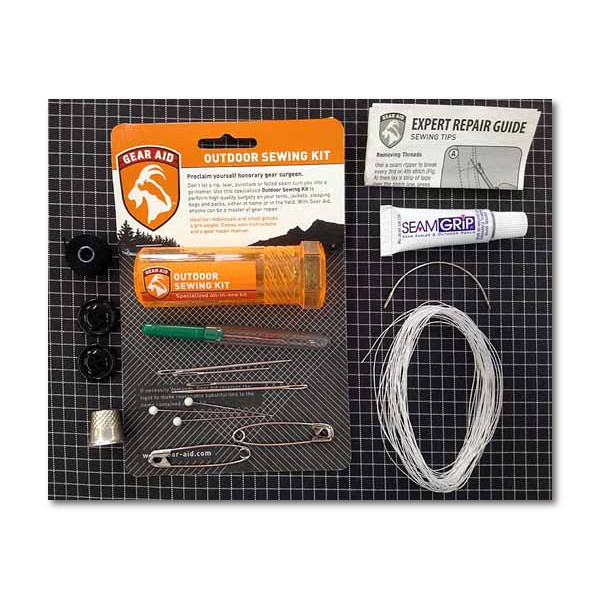This image features an outdoor sewing kit displayed on a black surface with a white grid pattern. At the center of the image, there's a bubble package with an orange banner reading "Outdoor Sewing Kit" and an orange shield featuring the Gear Aid logo, which includes a white silhouette of a goat. Inside the blister pack, there's an orange container labeled "Outdoor Sewing Kit," along with several needles, safety pins, an end picker, a roll of white thread, and some black, unidentifiable objects. 

To the right of the blister pack, there is a folded set of instructions titled "Expert Repair Guide, Sewing Tips." Below these instructions, there is a white tube with purple lettering labeled "Seam Grip" and an oval-shaped roll of thread. Additionally, there are some snaps and a silver thimble included in the set.